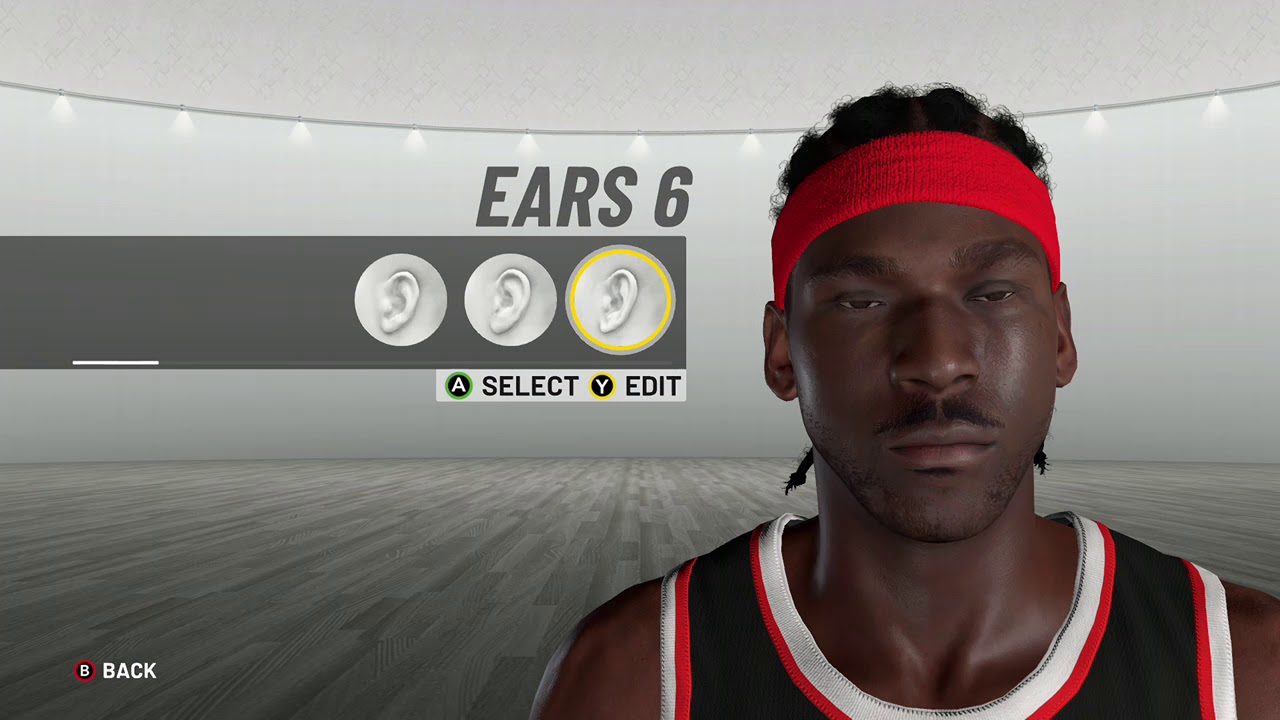In the image, a player is deeply immersed in a basketball video game, specifically in the character creation mode. The character being customized is a Black man with frizzy hair that appears to be in cornrows or previously styled as such. He is adorned with a bandana and wearing a predominantly black jersey with red and white trim. Currently, the player is fine-tuning the ears of the character, selecting from various options. The chosen ears are tall, narrow, and have pointy lobes, contributing to the realistic portrayal of the character. The character has dark skin that reflects light subtly, and his facial features include resting eyes that almost appear closed, and a mustache. The customization takes place in a setting that resembles a basketball court, devoid of hoops. The environment is characterized by wooden floors and an abundance of grey, with grey walls and ceilings, adding to the immersive atmosphere of the game.